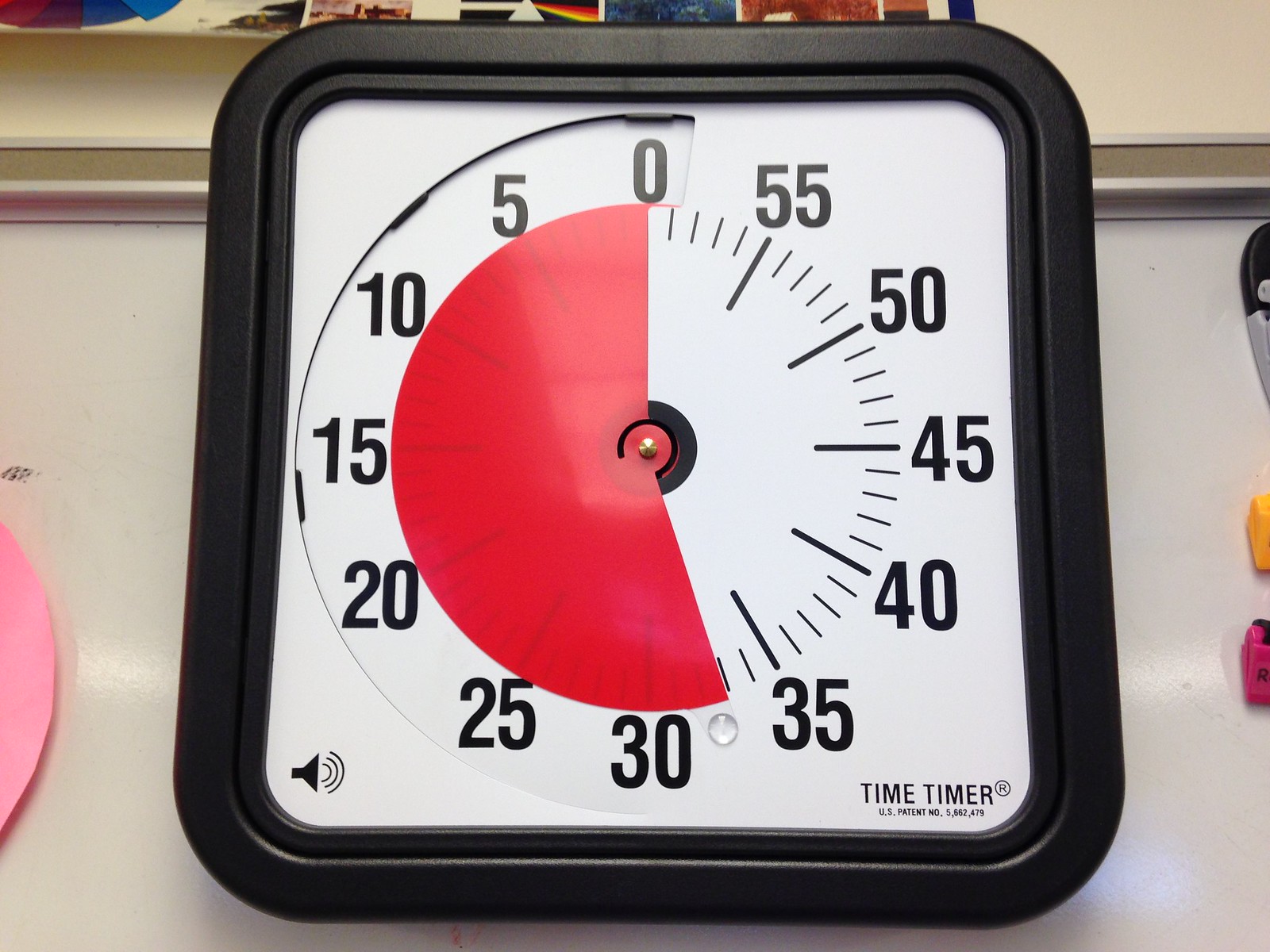This image features a large countdown timer with a robust black plastic frame that is roughly an inch thick and has smoothly rounded edges. The timer's face is a contrasting bright white, accentuating the clear, black numbers arranged in a clockwise direction, marked from 0, 5, 10, 15, 20, 25, 30, 35, 40, 45, 50, 55, and back to 0. Each number is separated by precise tick marks. A vibrant pink half-circle segment visually represents the time elapsed, stretching from the 0-minute mark to the 30-minute mark. In the bottom right corner of the timer's face, the text "TIME TIMER U.S. PATENT NUMBER" is printed in black, lending a touch of authenticity and branding to the device.